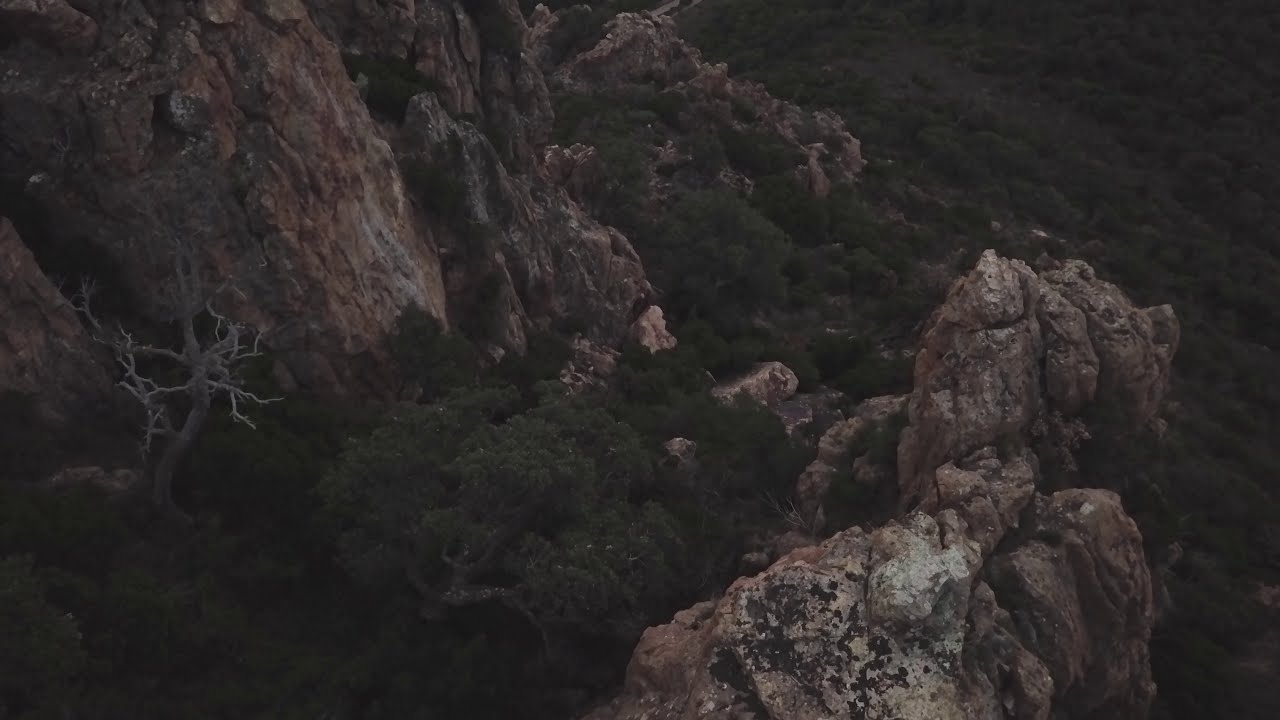The image is a high-angle shot, possibly taken from a drone or during a mountain hike, capturing a rugged and dramatic landscape. The scene features prominent rocky cliffs and jagged mountain sides, with sharp stone formations shooting upwards, predominantly in tan, brown, white, and dark gray hues. Nestled within the nooks and valleys of these formidable rock walls, a dense sea of vibrant green foliage flourishes, punctuated by numerous trees and bushes. Notably, one large, leafless tree stands out among the greenery, clinging to the side of the cliff. The overall atmosphere appears overcast, lending a murky, grayish tint to the scene, although under better lighting conditions, the green landscape would likely appear even more lush and vivid. This captivating view provides a bird's-eye perspective of the natural beauty and ruggedness of the mountainous terrain below.